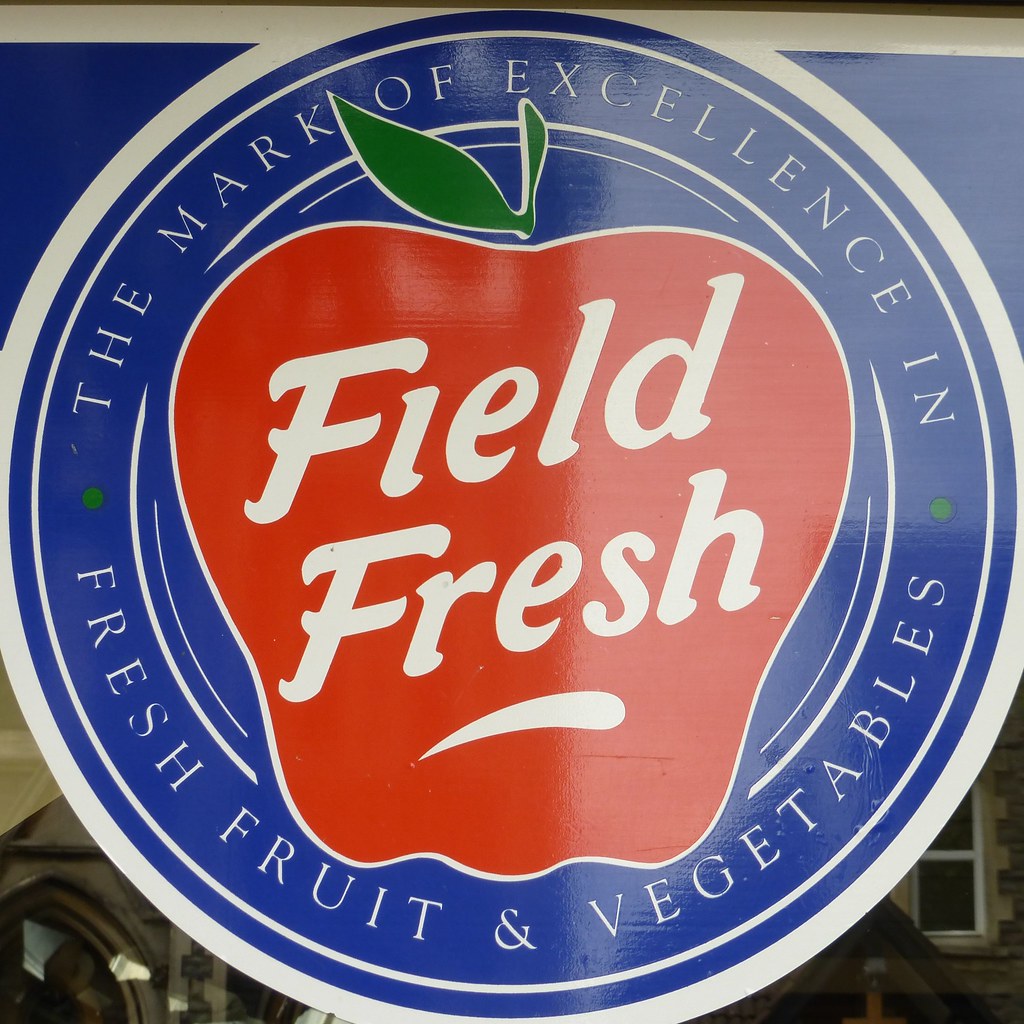The logo is circular with a prominent white outline and is filled with blue inside this outline. Within the blue field, there's a secondary white circle containing the text "The Mark of Excellence in Fresh Fruit and Vegetables" written around its perimeter. Positioned at the center of the logo is a large red fruit, resembling either a tomato or an apple, with a green leaf and stem on top. Across the red fruit, in white letters, is the phrase "FIELD FRESH," where "Fresh" is underlined. The design includes additional blue areas at the top left and right corners within the primary white outline. The overall composition combines multiple detailed elements to emphasize quality and freshness.